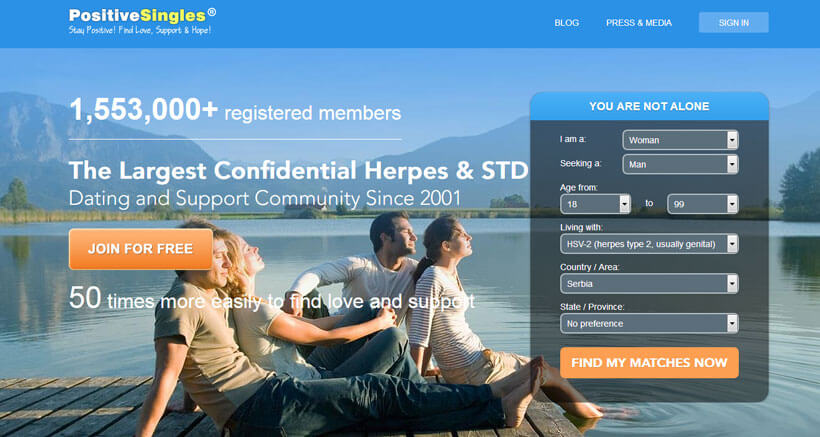This image appears to be a screenshot of the sign-in page for "Positive Singles," a dating website designed specifically for individuals living with herpes and other STDs. The page features a predominantly blue background and displays the slogan "Stay Positive, Find Love, Support, and Hope" prominently at the top. Below this, two couples are shown snugly seated together on a lakeside dock, creating a cozy and supportive atmosphere.

Above the couples, the text states, "1,553,000+ registered members," followed by a divider line, and then declares, "The largest confidential herpes and STD dating and support community since 2001." An orange button labeled "Join for Free" invites new users to sign up. Beneath this call-to-action, in white lettering, it states, "50 times more easily to find love and support."

To the right, a registration form is visible. It is headed by the reassurance, "You are not alone." The form includes several dropdown menus:

- "I am a:" with "Woman" as the default selection.
- "Seeking a:" with "Man" as the default selection.
- "Age from:" with a range from 18 to 99.
- "Living with:" defaulted to "HSV-2" (herpes type 2, usually genital).
- "Country/Area:" defaulted to "Serbia."
- "State/Province:" defaulted to "No preference."

At the bottom of the form, a green button labeled "Find My Matches Now" is ready for users to start their journey in finding companionship and support.